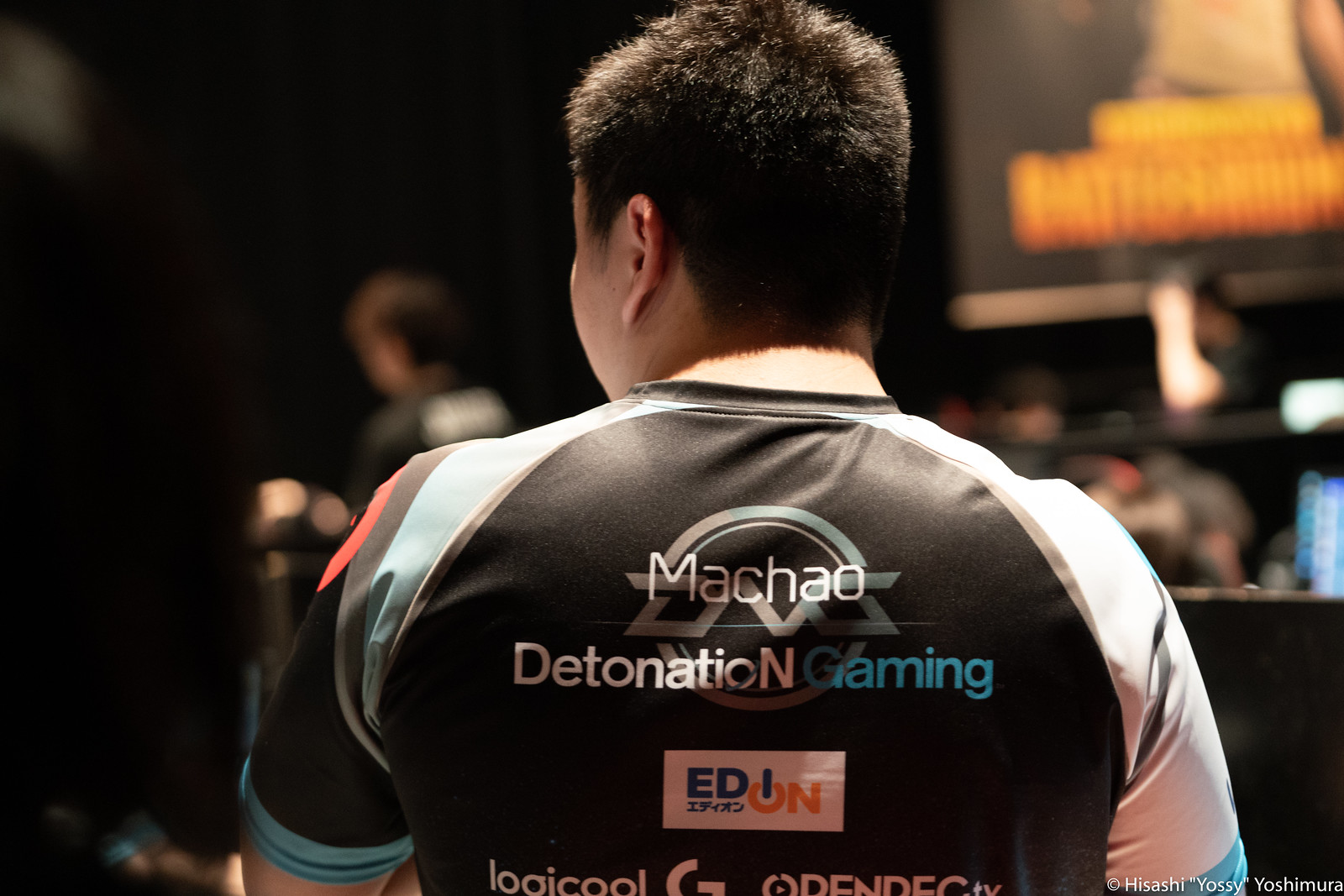This indoor photograph features a man with short, dark brown hair styled in a buzz cut. He is at the center of the image, with his back facing the camera, and his head slightly turned to the left, gazing off into the distance. He is wearing a black short-sleeved shirt with white accents on the sleeves. The back of his shirt is adorned with the text "Macho Detonation Gaming," with "Detonation" notably ending with a capital 'N.' Below this text, a logo reads "ED ON" in a distinctive white rectangle with "ON" highlighted in an orange font. Further down, there's additional text that says "Logicool G Odin Deck TV." 

In the lower right corner of the image, there is a small copyright notice: "Hisashi Yoshimura," suggesting the photographer or possibly indicating the man's name. The setting appears to be a dimly lit area, possibly a bar, auditorium, or gaming convention, indicated by the blurry figures in the background and a banner in the upper right corner. The ambiance suggests an event or social gathering dedicated to gaming, with the man possibly watching something or someone to the left, likely a presentation or competition, given the context and his focused posture.